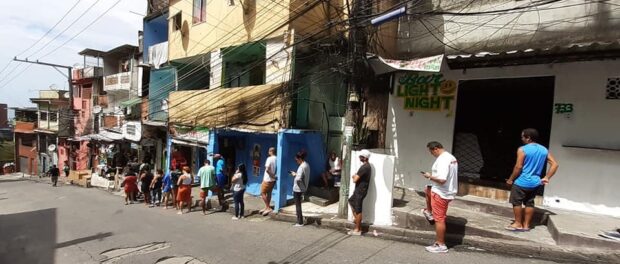A photograph depicts a narrow, worn-down street lined with small, cement buildings of various colors, including blue, pink, white, and yellow, suggesting a scene possibly somewhere in Mexico. The structures appear dilapidated, lacking doors and windows, and have uneven signage. Running parallel to the street are wooden planks, and the surface is marked by numerous chipped areas and potholes. A queue of people, many in shorts, stands along the sidewalk and the edge of the street, under a hot climate. Electric cables hang precariously low above the street, reachable by jumping. On the right side, the visible building features text that reads "light at night" followed by the address "723". The overall ambiance of the area reflects a struggling, impoverished neighborhood with a third-world atmosphere.